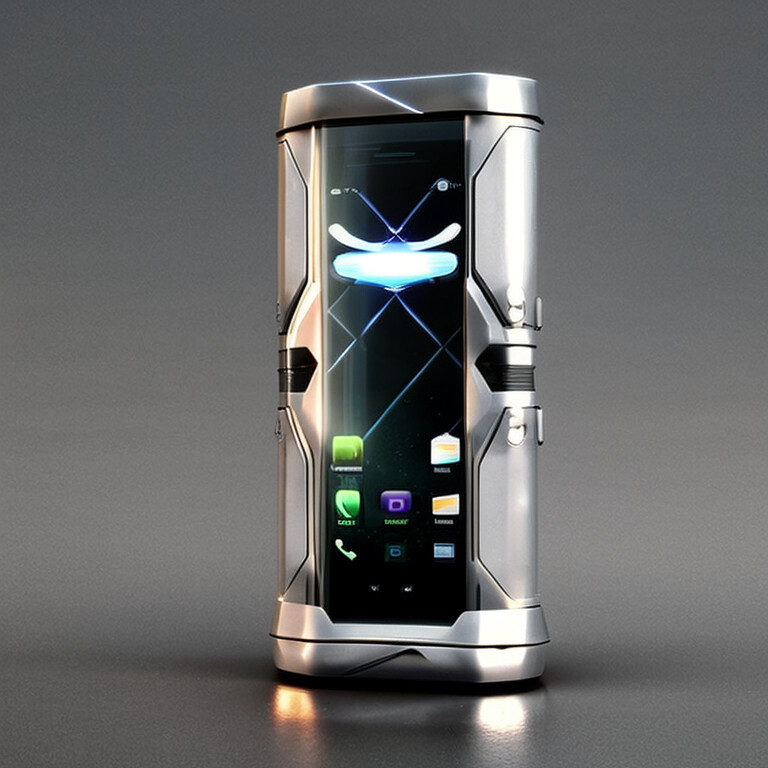The image is a highly detailed color photograph showcasing a futuristic cell phone or smartphone positioned upright at the center against a dark gray or black background. The main body of this device appears to be a sleek, silver-colored box with a reflective surface, casting a soft glow of yellow and white lights on the surface below. The phone's interface, which is somewhat reminiscent of current models but with a distinctly sci-fi design, features a black display panel with a striking blue, butterfly-like design at the top. The panel is adorned with several squared icons in green, purple, and white, with a prominent call button located at the bottom left. Hovering above is a luminous, turquoise-colored object adding to the futuristic aesthetic. The entire setting exudes a high-tech gadget vibe, accentuated by the subtle reflections and the advanced, computer-generated look of the scene.